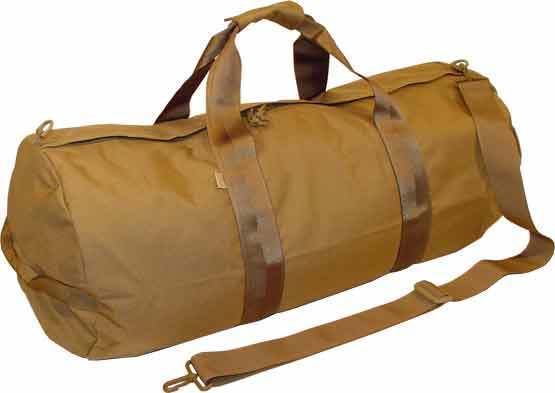This photograph features a rectangular, horizontally-aligned duffel bag in a medium brown color, crafted from what appears to be a waterproof nylon material. The bag is detailed with darker brown handles, which have a Velcro strap in the middle to hold them together. These handles, thick enough to remain upright, hover above the bag rather than resting against it. A shoulder strap, dangling unattached on one side, lies on the ground to the right. Prominent clips on either side of the bag are meant for strap attachment. The duffel bag, slightly elongated compared to average sports bags, has a tiny light yellow tag whose brand or text is indiscernible. The entire composition is set against a stark white background, showcasing the bag's side profile view from left to right.